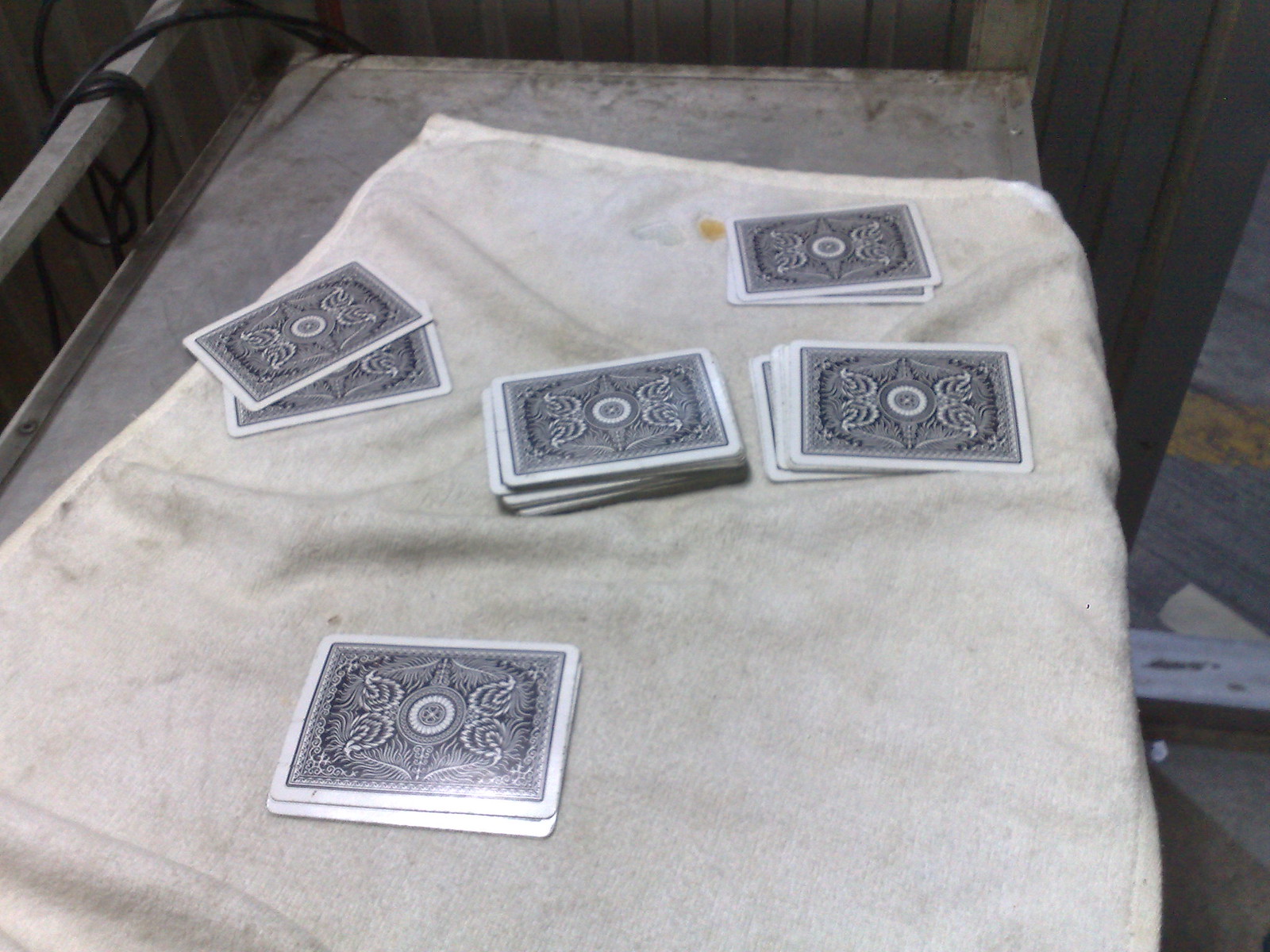The image depicts a metal table or shelving unit that is partially covered by a heavily soiled towel, which appears to have once been white but is now a grimy gray-black with visible yellow stains. The towel is not fully stretched out across the surface, revealing parts of the metal beneath. Arranged on the surface are several small stacks of playing cards. Two cards sit on one side, another pair is positioned opposite, with the bulk of the deck in the middle. Additionally, there are about twelve cards spread away from the main deck and another two cards oriented towards the viewer.

The playing cards have a patterned design with blue and white colors and standard card symbols in the center. There are no people present in the image, but the card arrangement suggests a paused game, as if someone had been dealing cards but had to leave abruptly. In the background, a coiled piece of cord is wrapped around an edge of the metal structure, further adding to the disorganized and abandoned atmosphere of the scene.